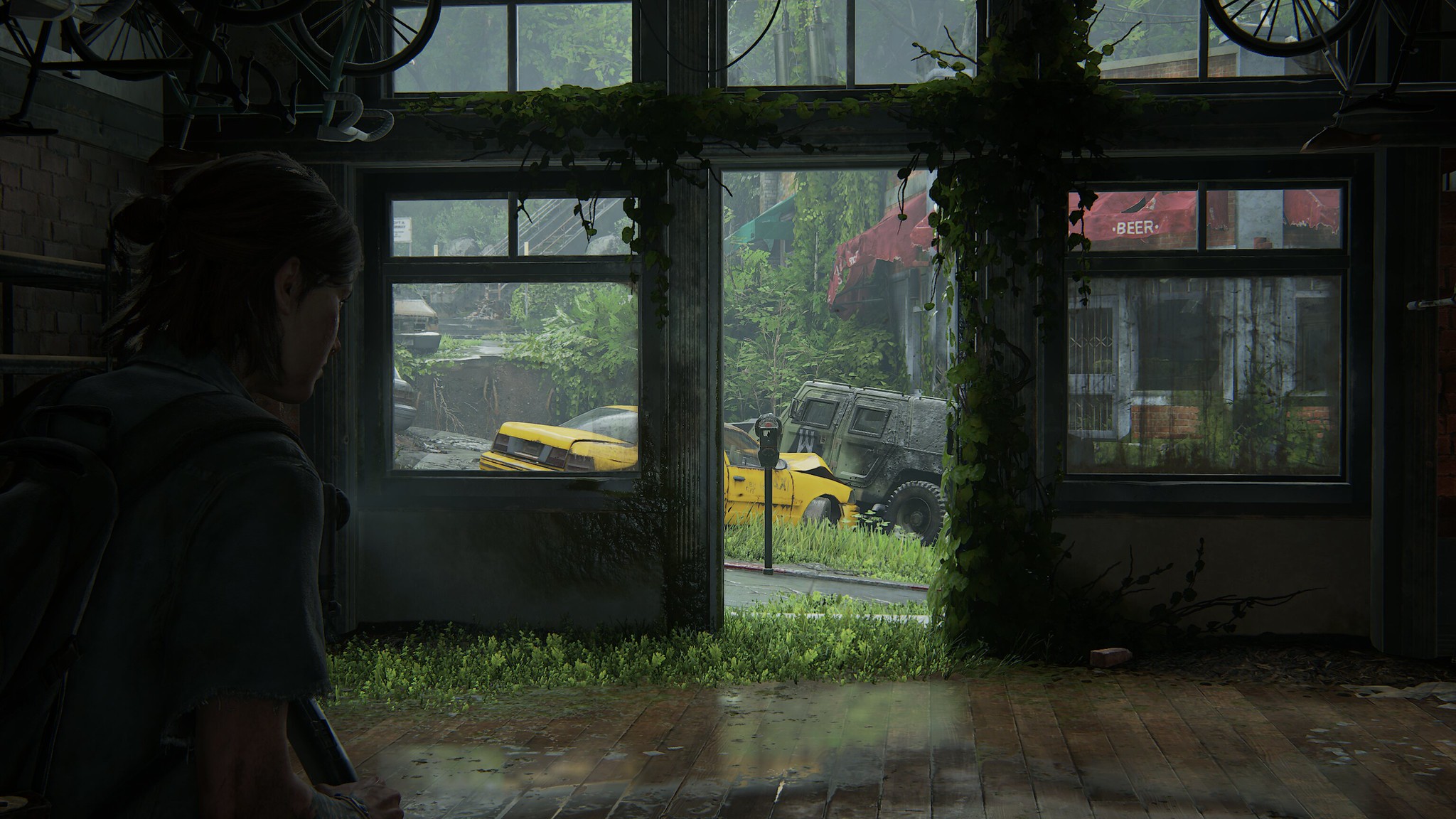The image appears to be a highly realistic screenshot from a video game, likely from "The Last of Us," featuring a meticulously detailed indoor scene. The setting is inside a dilapidated building with ivy cascading down the walls and spanning onto the shiny, possibly wet, wooden or brick-colored floor. Prominently, on the left side, stands a character named Ellie, identifiable by her shoulder-length black hair, short-sleeved gray shirt, and backpack. The building's interior also features curious greenery sprouting from the floor. In the center, an open door is flanked by two see-through windows revealing an outside street scene, suggesting rain with its wet reflections. Outside, a yellow taxi with a crumpled hood and a gray Humvee-like vehicle are parked, indicating a state of disrepair. Across the street, a storefront with red awnings bearing the white word "Beer" can be seen, along with overgrown plants and bushes, hinting at an overall sense of abandonment and decay.